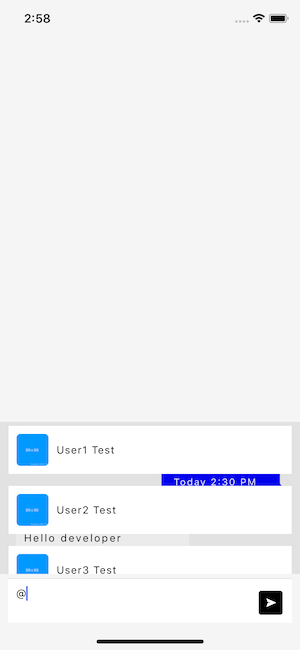The image is a screenshot taken from a mobile phone, indicated by the time display of "2:58" in black text at the top of the screen. The background is a light gray color throughout. At the top, there are three horizontal dots on the left, presumably a menu option, followed by the Wi-Fi symbol, and a fully charged battery icon represented by a solid black strip.

The midsection of the screen is completely empty, displaying only the gray background. Near the bottom of the screen, there are three user inputs labeled "user one test," "user test two," and "user test three." These entries are in a muted grayish-black color. Each user input is followed by a small blue square containing an almost indistinguishable white symbol or text, possibly tiny characters or plus signs.

At the bottom of the screen, an input box shows the user beginning to type the "@" symbol. There is also a send button represented by a black square with a right-facing arrow, ready for use.